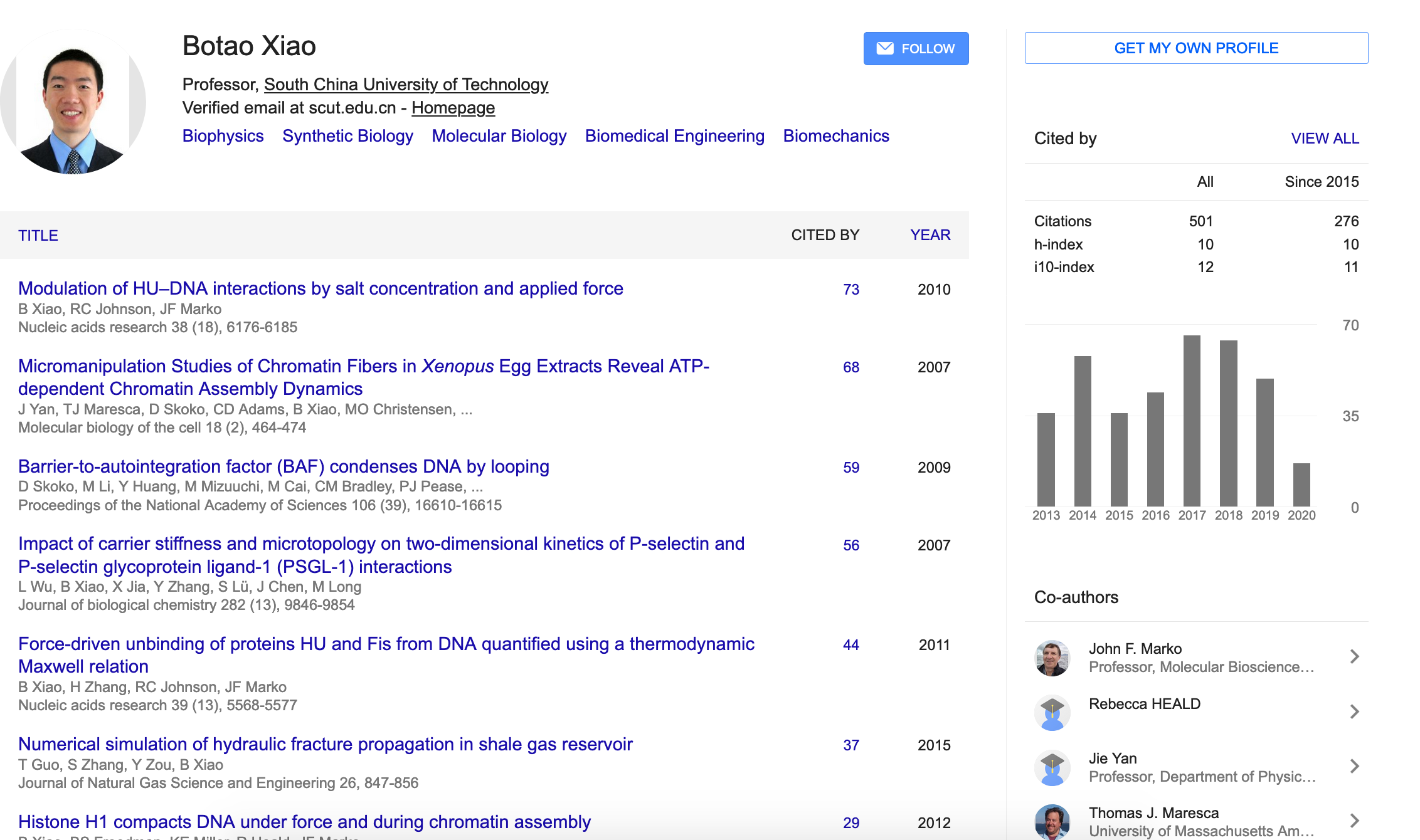The rectangular image features a detailed academic profile. The long side of the rectangle runs from left to right. On the far left, encased in a circular frame, is a profile picture of an Asian man. Above the image, it is indicated that he is a professor at the South China University of Technology. Directly below, there is a mention of a verified email at "scut," followed by terminology such as "homepage," "biophysics," "synthetic biology," "molecular biology," "biomedical engineering," and "biomechanics." 

A blue box containing a white envelope icon and the word "Follow" in white letters is prominently displayed in this section.

On the right-hand side of the image, a vertical column features the text "Get my own profile." Below this, it reads "Cited by" with an option to "View all citations." The citations tally up to 501. Further below, it lists the h-index at 10 and the i10-index at 12. Adjacent to these statistics is a bar graph, likely representing the citation data.

Below the bar graph, there is a list of co-authors, including names like John F. Marco, a professor of molecular bioscience, among others. On the left side of this section, the word "Title" appears, followed by a series of article titles highlighted in blue, indicating they are hyperlinks. Next to each article, there is a "Cited by" column displaying the number of citations each article has received, along with the corresponding years.